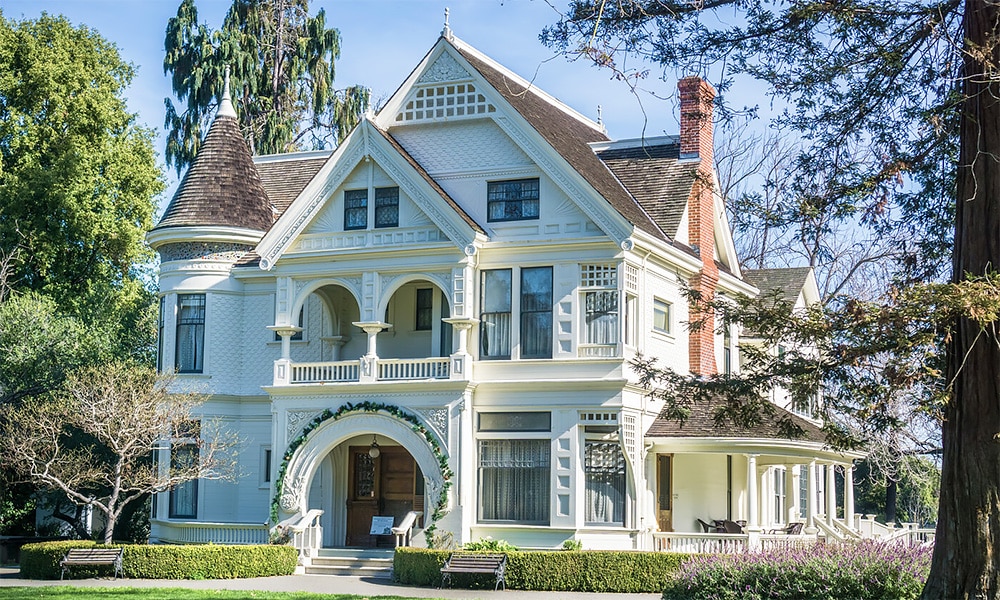This photograph captures a grand and elaborate old Victorian-style home, predominantly white with a gray roof and a prominent reddish brick chimney on the right side. The house stands three stories tall and showcases a variety of intricate architectural details. At the center of the front facade, there is a grand archway flanked by stairs that lead up to two large brown wooden doors, with vines adorning a white arch above them. One door features a window, and two benches flank the entrance, nestled against well-manicured hedgerows.

On the second floor, directly above the large entryway, a spacious balcony or veranda is supported by three pillars and offers a picturesque view of the front lawn. The balcony and the surrounding patio areas, including a sun porch equipped with furniture, provide additional open-air sitting areas, emphasizing the home's elegance and luxury. The home’s front features various window designs, including two smaller windows under a steeple on the left side and additional windows of varying sizes scattered symmetrically across the structure aligned both vertically and horizontally.

The extensive grounds are immaculately landscaped, with a variety of trees and bushes enhancing the home’s lush surroundings. Weeping willows are particularly prominent, contributing to a serene, genteel atmosphere. A large lawn extends in front of the house, and a dense concentration of trees sits to the right and left of the home, including a prominent tree at the forefront of the image. The overall scene, captured in daylight, emphasizes the home's majestic presence and its substantial, visually stunning grounds. This exquisite home exudes an aura of sophistication and stately Southern charm.